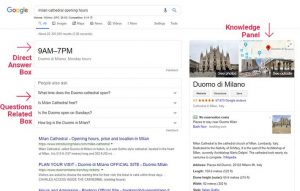The image appears to be a screenshot from Google, displaying various features of a search results page. On the left side, the distinctive colorful Google logo is visible in the upper left corner, accompanied by the search bar. Although the exact search query is unclear due to tiny font size, below the search bar, there is a prominent search result in bolded text reading "9 a.m. to 7 p.m." A red arrow with the label "direct answer box" points to this result.

Further down, the "People also ask" section is highlighted, featuring a red font and another red arrow labeled "questions related box," although the small text is unreadable. 

On the right side of the image, there appears to be a visual representation of a knowledge panel. This includes several pictures depicting what seems to be a museum or historical building. Above these images, a red font with an arrow pointing downwards labels this section as the "knowledge panel," which also includes a title that looks like it might be an Italian name for the structure.